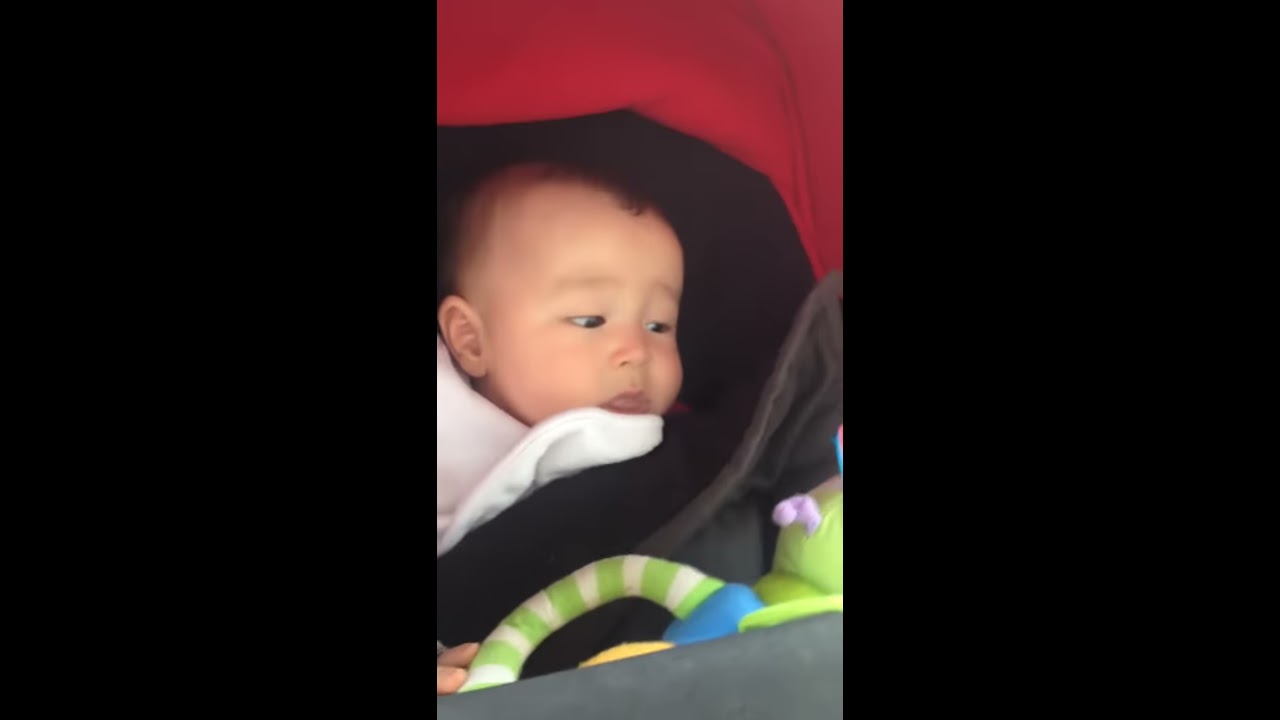A detailed photograph captures a small Asian baby, around eight months old, swaddled in a black blanket and positioned in what appears to be a car seat or cradle. The baby has fine dark brown hair, with a noticeable tuft towards the front and curious, slightly slanted dark brown eyes looking off to the right side of the image. Above the baby, there's a red pillow or fabric, and the baby is resting against a raised black and white striped handle that seems part of the carrier. In front, scattered around the baby, are some toys, including a distinct green and white striped alien-like toy with a blue torso and a green head, which seems to have caught the baby's serious gaze. The baby, despite the serious and curious expression, has a slightly pouty look on his face, appearing both fascinated and on the verge of sleep. The overall photo is framed with black bars on both the left and right sides, drawing focus to the baby swaddled comfortably in the center. The dominant colors in the image are black, red, white, green, blue, and gray, creating a vibrant and detailed setting focused entirely on the baby.